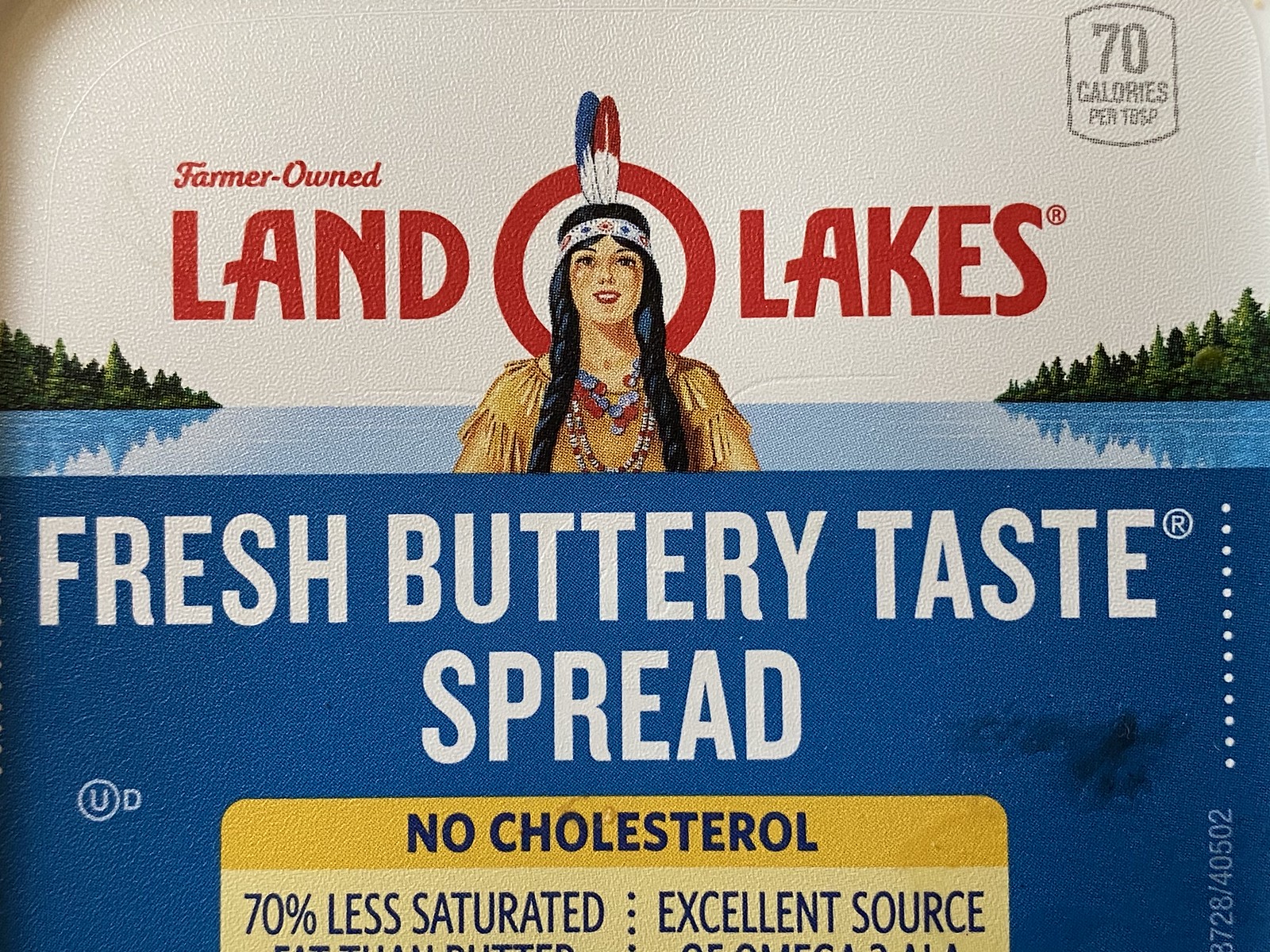The image is a detailed, up-close view of a vintage Land O'Lakes product label. The label prominently features "Farmer-Owned Land O'Lakes" written in red at the top. The center highlights an illustrated Native American woman with long black hair in two braids. She wears a headband with one red and one blue feather, traditional leather buckskin clothing, and beaded necklaces. Behind her, a serene blue lake reflects the sloping forested hills on either side, adding a tranquil backdrop. Below the image, a blue section with white text reads "Fresh, buttery taste spread." Adjacent details mention "No cholesterol" and "70% less saturated," with some portions of text partially obscured. The sky in the background is depicted as a white, blank space. A small text above "Land O'Lakes" notes "Farmer-Owned," emphasizing the cooperative nature of the brand.